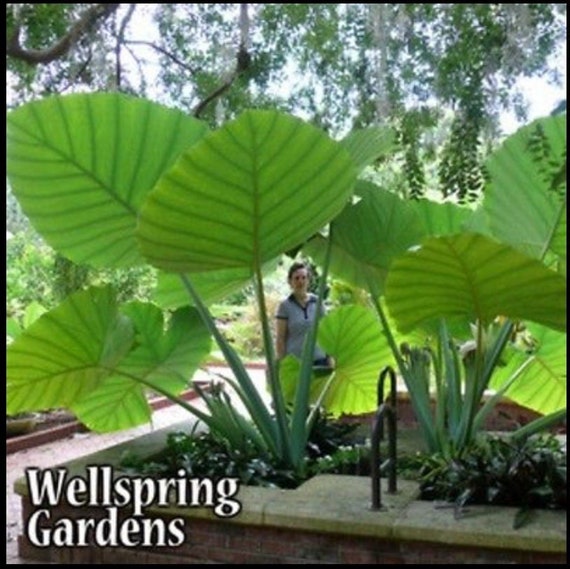In this vibrant outdoor advertisement for Well Springs Gardens, a stunning display of colossal green plants dominates the foreground, their enormous elliptical leaves creating an impressive visual impact. These verdant giants, which resemble burdock roots or hosta plants, sprout from a meticulously crafted brick-raised flower bed topped with a flat stone ledge. The scene is framed within a square, four-inch photograph bordered by a thin black outline. 

In the lower left corner, the garden's name, "Wellspring Gardens," is prominently featured in bold white print with a black outline. Amongst the lush greenery, a person of Caucasian descent is visible in the central background, their features obscured but their presence adding depth to the image. They wear a short-sleeve shirt, which appears blue or gray, blending naturally into the serene setting. 

The background reveals a sunny day with a clear blue sky, towering trees, and strands of Spanish moss cascading down, suggesting the garden's proximity to a forest. The combination of the gigantic plants and the natural surroundings emphasizes the garden's grandeur and beauty, making it an alluring invitation to experience Well Springs Gardens.